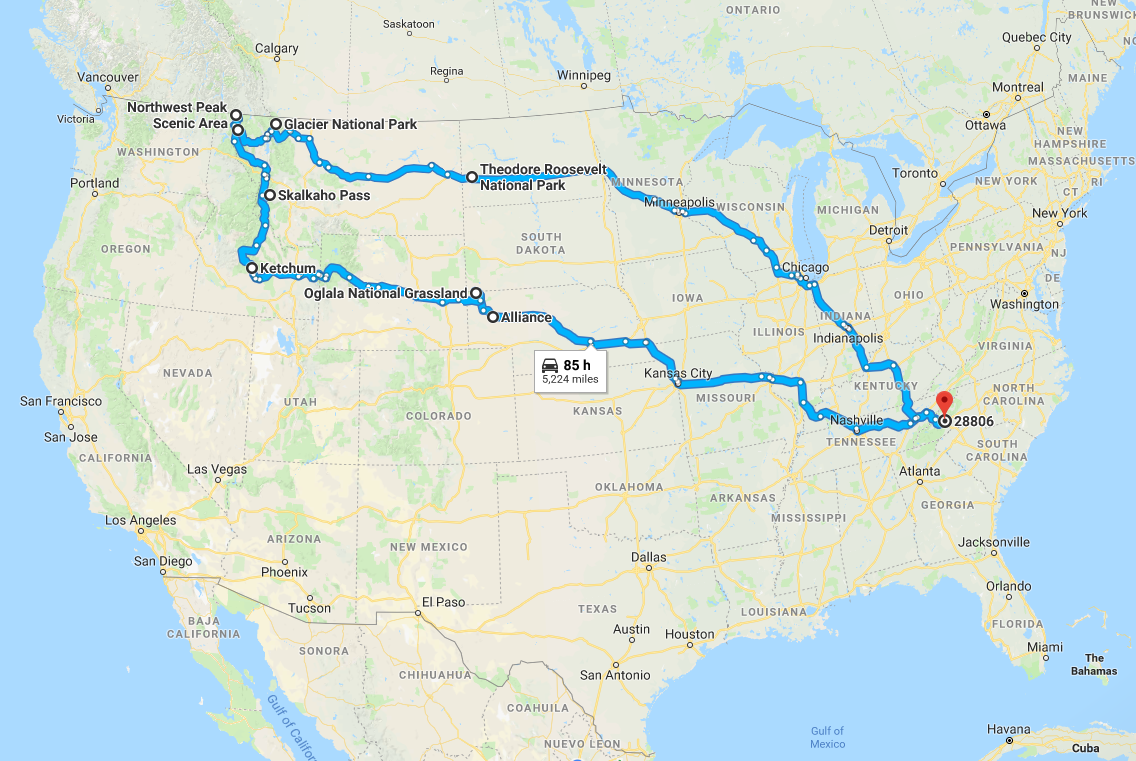This image displays a detailed Google Map of the United States, incorporating visible sections of Mexico and Canada. The terrain is depicted in light green with darker green hues indicating dense areas, accompanied by yellow roads and surrounding bodies of water in blue. Central to the image is a prominently marked blue route showcasing a planned road trip.

The journey initiates from zip code 28802 in Tennessee, identified with a red location marker within a small black circle. The route forms an extensive loop covering various states and key landmarks. It heads north through Kentucky and Illinois, passing through Chicago and Minneapolis before reaching Theodore Roosevelt National Park. From there, it continues to Glacier, near the Canadian border at the top of Idaho. 

The route then loops back down through Ketchum, Idaho, and Alliance, moving southward through Kansas City and finally returning to Nashville, Tennessee. The entire trip covers approximately 5224 miles and culminates at the northwest peak scenic area. Throughout the map, the journey is clearly highlighted, providing a comprehensive visual guide of the extensive road trip.